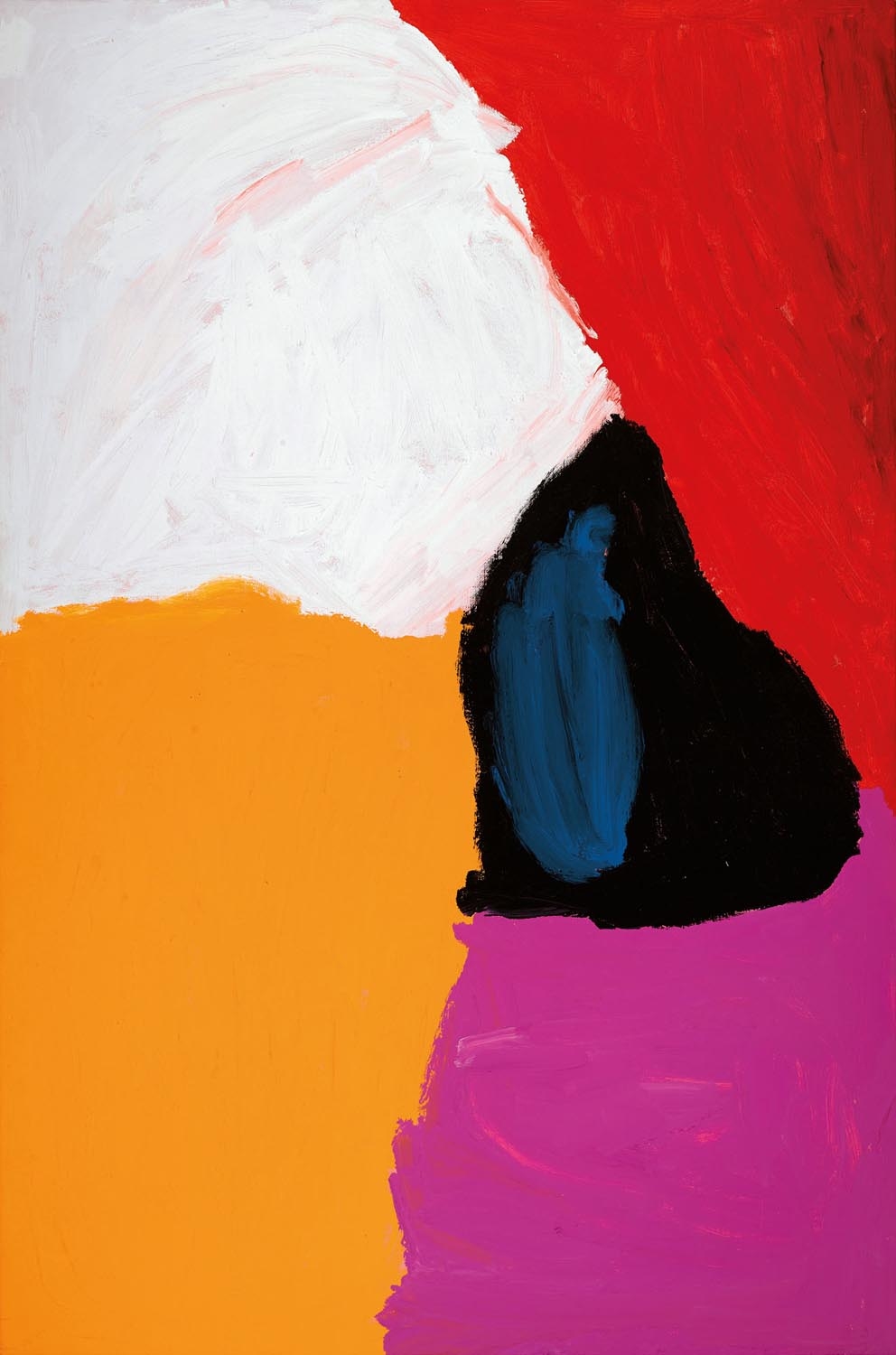The vertical rectangular painting is a vivid abstract composition characterized by its distinct sections of color and shapes. The top left part of the painting is predominantly white, interspersed with faint pink or red lines. Adjacent to this, in the upper right section, is a dark red area with visible lighter red streaks. Dominating the center of the image is an irregular black shape, resembling a mix between a triangle and a circle, with smears of blue or cerulean paint overlaying it. The lower half of the painting is divided into two primary sections: the bottom right showcases a purple hue, with streaks of pink woven in, while the lower left corner features a solid, bright orange block resembling a rectangle. The overall arrangement creates a stark contrast between the white and red at the top and the orange and purple at the bottom, accentuated by the central black and blue form.